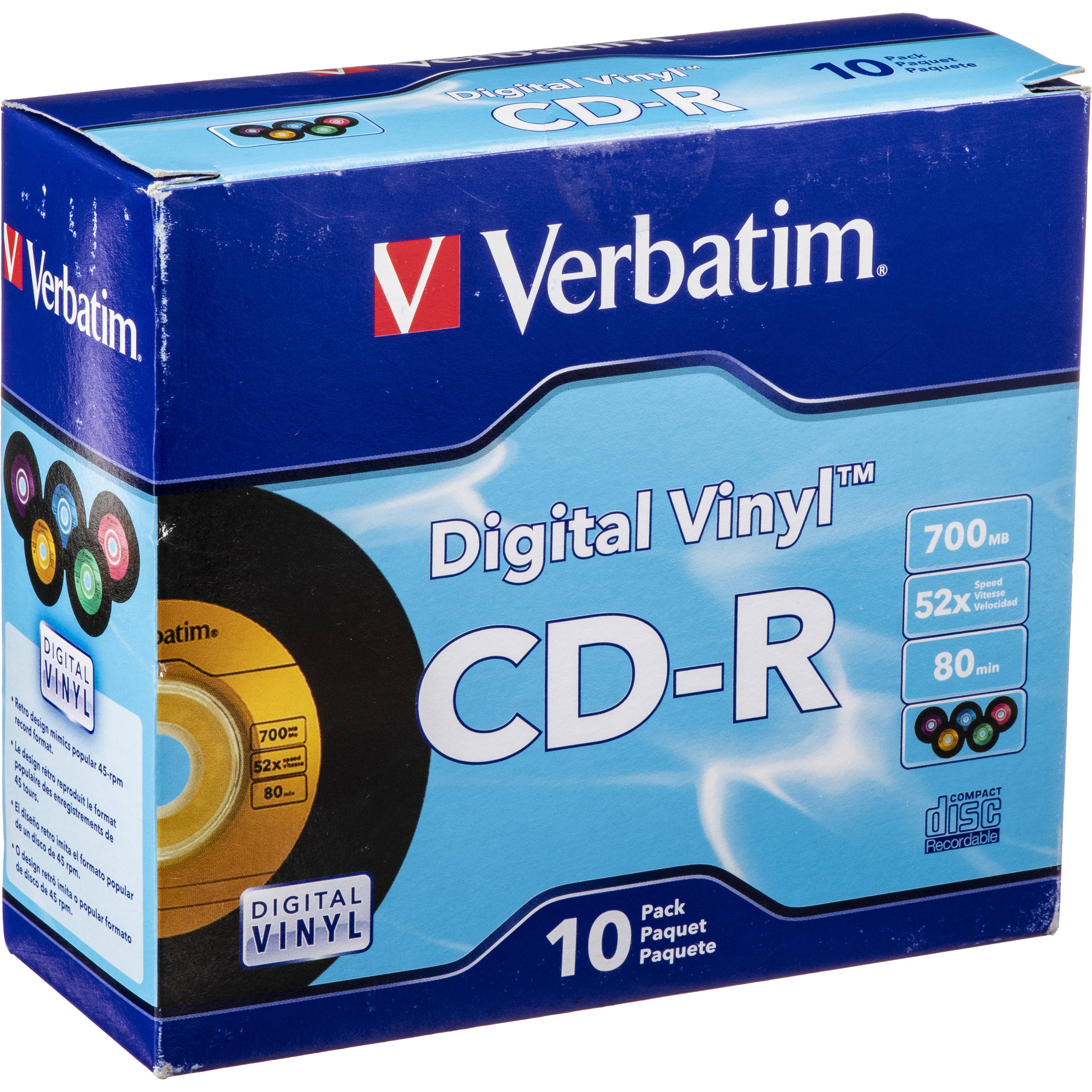This image showcases a 10-pack product box of Verbatim brand digital vinyl CD-Rs, designed to mimic the look of old vinyl records with a black border replacing the reflective laser. The predominantly blue box features a dark blue top and bottom section and a light blue middle with white smoke effects. The Verbatim name, displayed in white lettering, is accompanied by a red square with a white 'V' on the dark blue section. The box front highlights various product details in white text, including "Digital Vinyl CD-R," "700 megabytes," "52x speed," and "80 minutes." Additionally, it shows an image of a black-and-gold label CD resembling a vintage vinyl record and a smaller picture showing the five colored discs included in the pack: purple, gold, blue, green, and red.